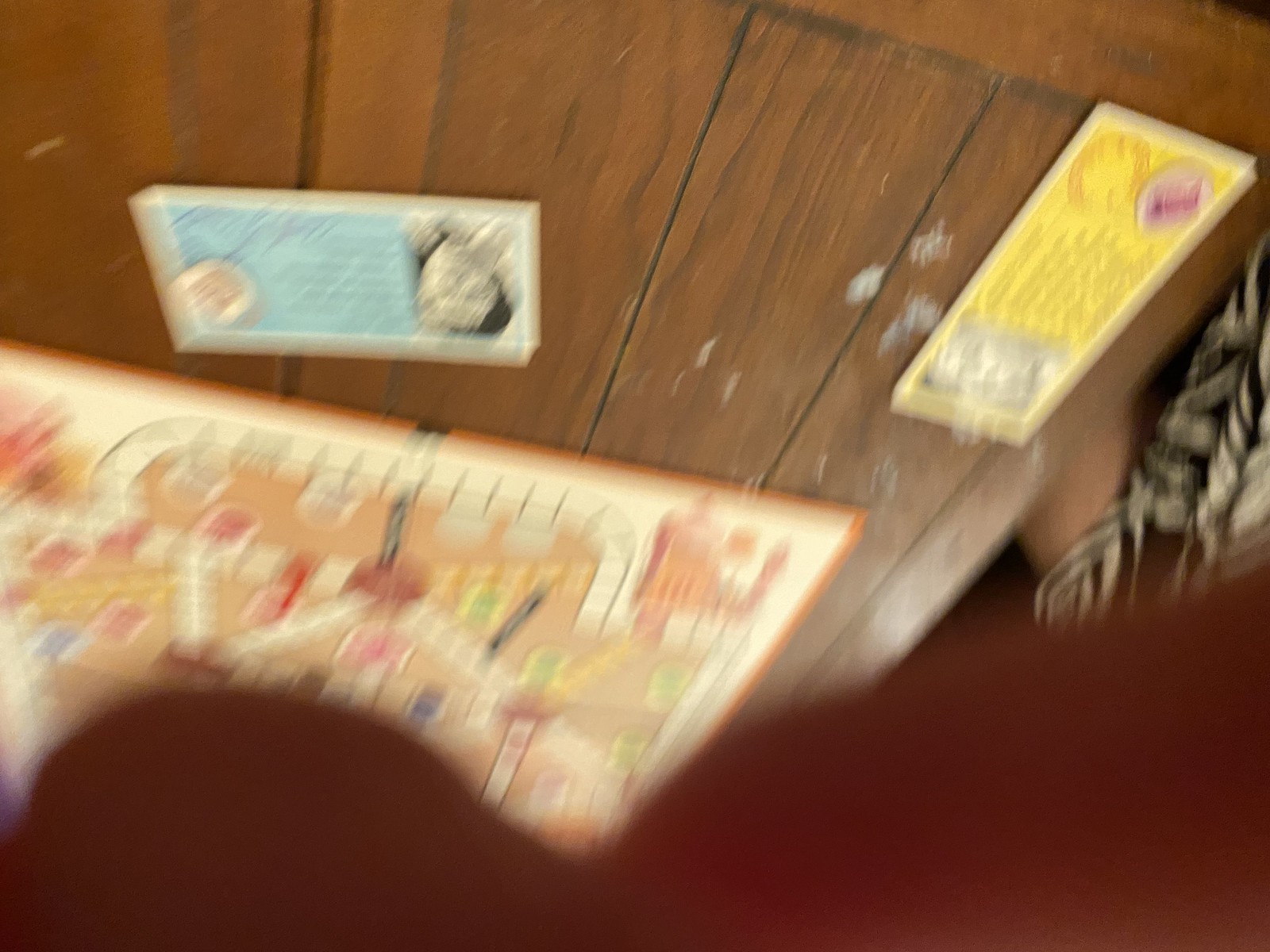The photograph appears to have been hastily taken without the photographer realizing, as evidenced by the presence of a hand or thumb intruding at the bottom edge of the image. Additionally, the image is upside down, out of focus, and not properly zoomed in, suggesting an impromptu shot. The scene captures a brownish table on which a board game is spread out. The exact game is unidentifiable due to the blurry nature of the photo, but it features a board and several small tiles evocative of games like Candyland, albeit with a predominantly brown color scheme. Scattered around the board are a few rectangular pieces of paper, possibly game-related items or paraphernalia.